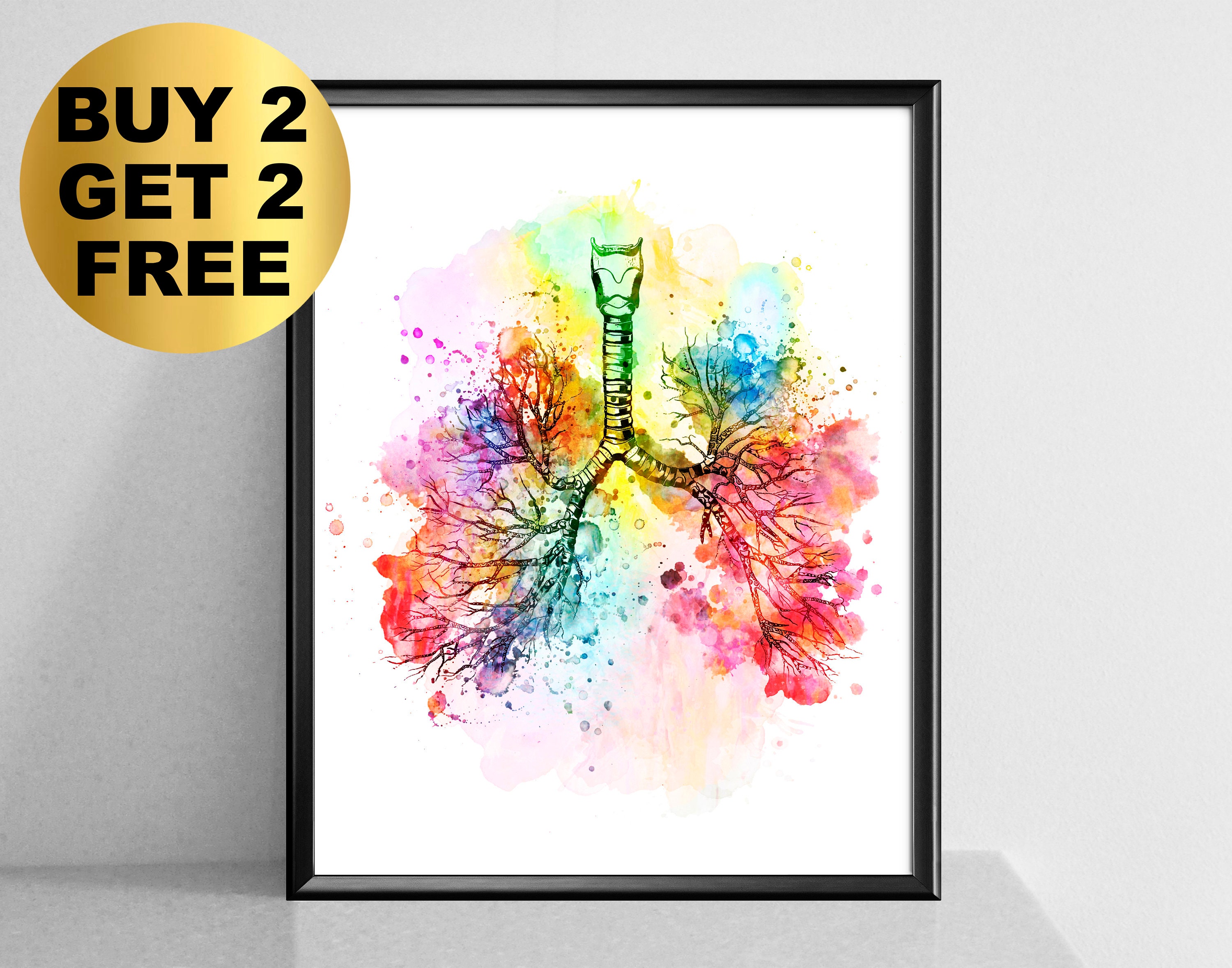The image features a framed artwork on a white tabletop background, predominantly showcasing a vivid portrayal of an anatomical structure resembling the bronchial tubes and airway of the lungs. The structure, branching out like a tree, is central to the composition and vividly adorned with splashes of various watercolors, including blue, purple, red, green, yellow, and orange. These colors suggest the locations of the lungs and spread out in an almost explosive pattern, adding to the visual intrigue. The black frame of the picture contrasts starkly with the white background, drawing attention to the central artwork. Notably, in the top left corner of the image, a gold circular sticker prominently displays the offer "Buy Two, Get Two Free," enhancing the commercial aspect and making it an eye-catching piece that might be seen in online retail spaces like Amazon.